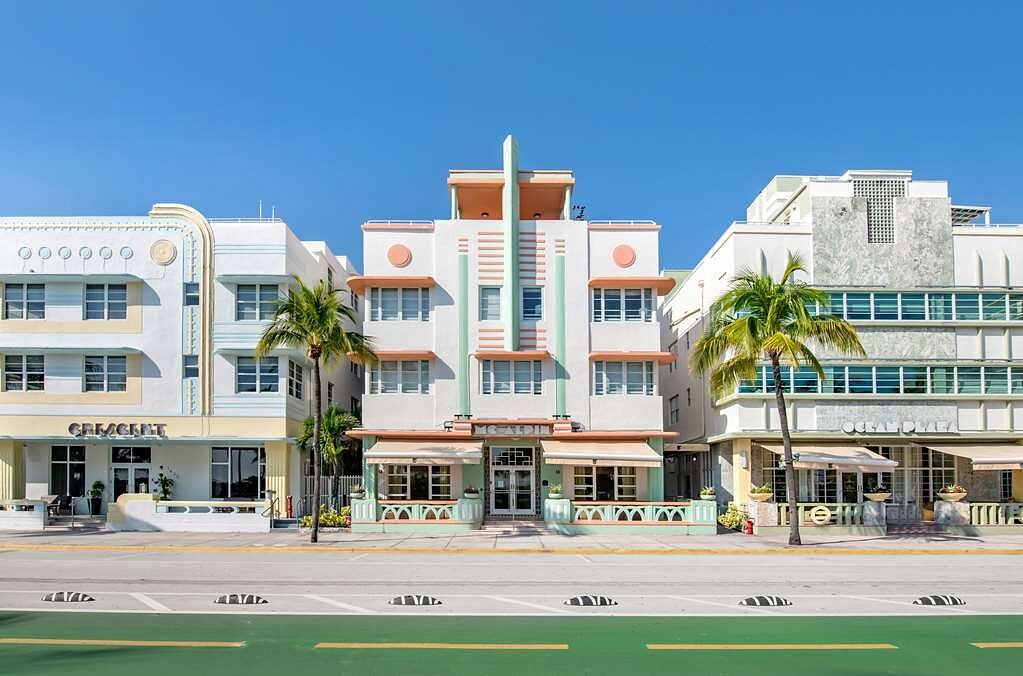The image showcases a vibrant street scene, likely in Miami, Florida, characterized by its striking Art Deco architecture and pastel colors. Dominating the foreground is a green street with a yellow line running down the center, flanked by a very light-colored sidewalk. Three distinct, squarish white buildings line the street, each adorned with its unique pastel trim.

On the left stands a three-story white building with light blue and peach trims, possibly housing shops on the ground level and apartments above. In the center, the focal building features light green façades with peach trimming and a sign that reads "McAlpine." This building also has a double-door entrance and a patio cover, ideal for shaded relaxation. The building to the right is another three-story white structure, this time with grey and light blue accents, and a balcony stretching across its width. This building prominently features a sign reading "Ocean Place" above its doors and appears to house a restaurant starting with a "G."

Two tall, vibrant palm trees stand in the center, adding to the tropical ambiance under a bright, cloudless blue sky. Little fence barricades are visible in front of each building, contributing to the organized, lively street atmosphere.